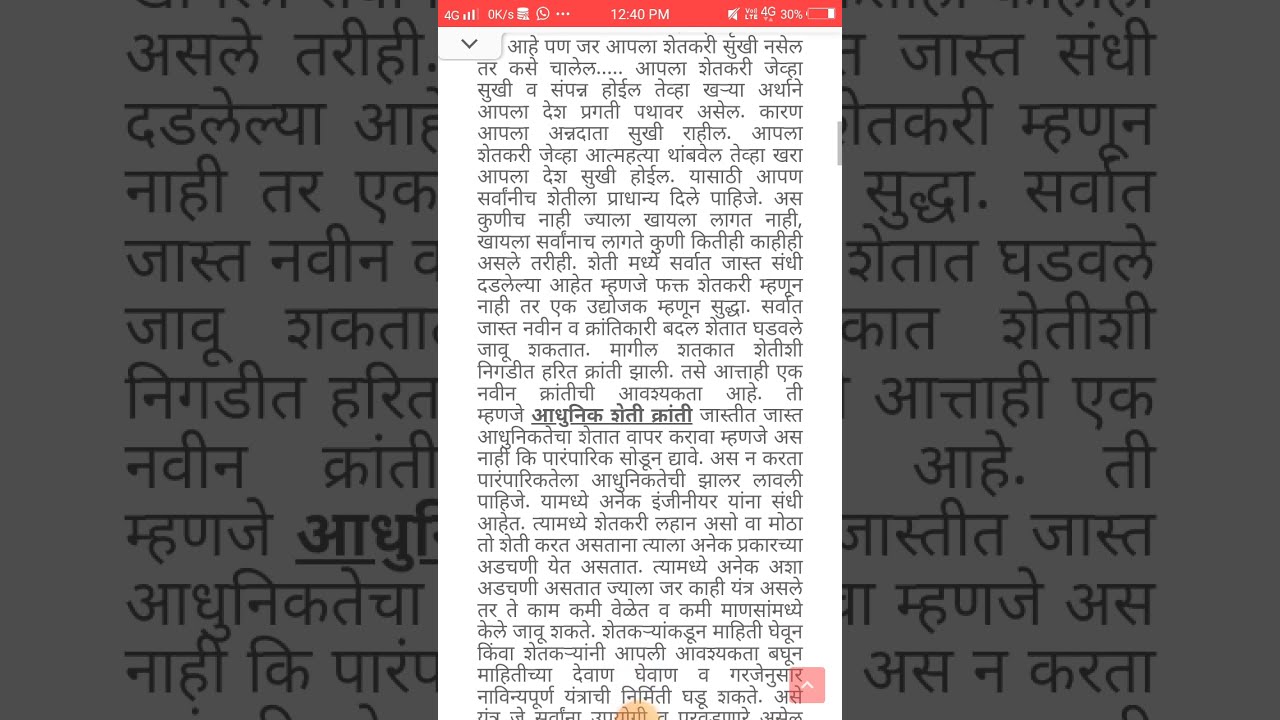The image is a horizontally extended screenshot of a smartphone displaying a lengthy block of text in a Southeast Asian script, though the exact language remains uncertain—it could be from regions such as India, Bangladesh, or neighboring countries. The text, in black characters, stands sharply against a white background. At the top of the screenshot, a red status bar shows various phone details: the time (12:40 p.m.), a 4G connection indicator, the signal strength, and a battery level at 30%. The screenshot appears to have been horizontally stretched, incorporating zoomed-in sections of the same text, making the script appear larger on the left and right sides of the image.